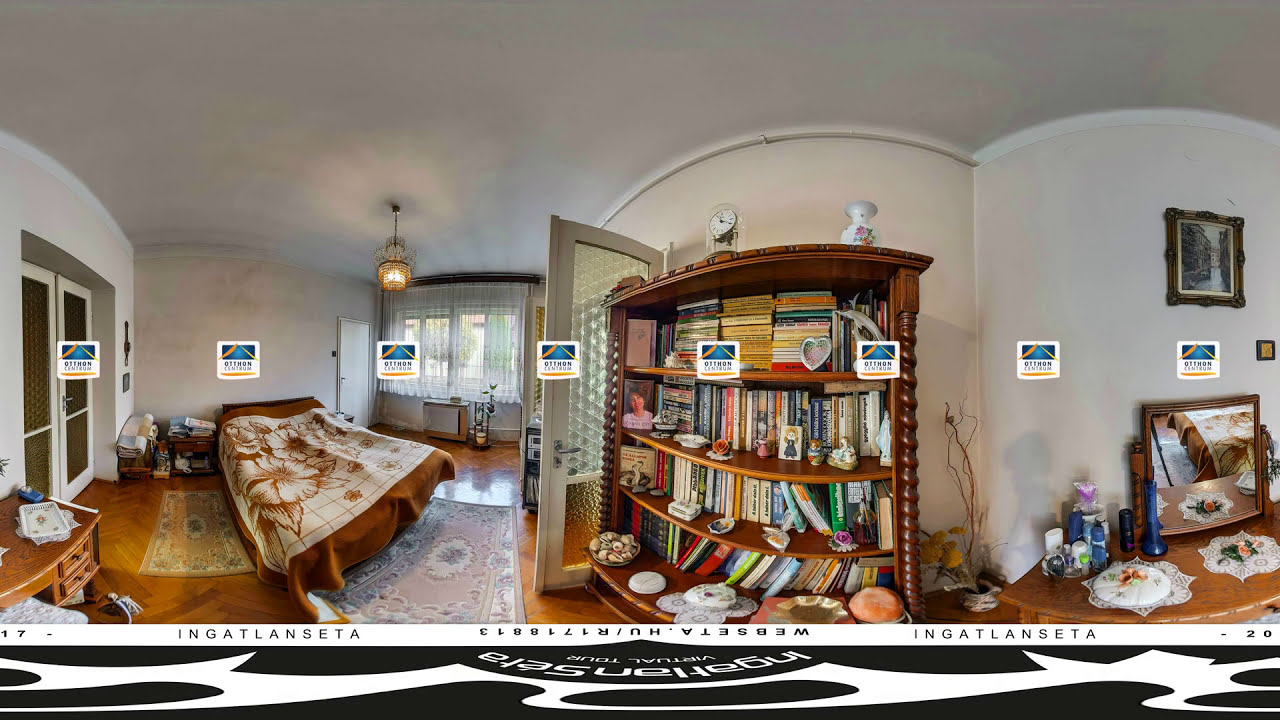The image showcases a panoramic view of a spacious bedroom, taken with a fisheye lens that exaggerates the room's dimensions and creates a slight distortion. The walls and ceiling are painted a crisp white, complementing the warm tones of the wood panel flooring. 

To the left of the room, there are two double doors with glass panels, adjacent to a small table. Nearby, a bed occupies the left corner, adorned with a combination of tan, rust-colored, and flower-patterned blankets, and sits atop an area rug. Behind the bed, a row of four windows allows ample natural light to flood the space. A door is situated between the bed and the windows.

Centered in the room is a large bookshelf brimming with books arranged both vertically and horizontally, along with various trinkets. Beside the bookshelf, towards the right, is a picture frame mounted on the wall above a side table that holds another picture and additional small items. Hanging from the ceiling is a chandelier, adding an element of elegance to the room. 

In the middle of the image, there's a distracting watermark with seven gold and blue logos and unreadable text, likely indicating the image is part of a virtual tour, possibly labeled "Webster Her" and "virtual tours." A desk with a mirror, covered with doilies and more trinkets, is positioned near the open door leading to the bookshelf.

Overall, the room is a blend of cozy and organized spaces, designed to be both functional and inviting.